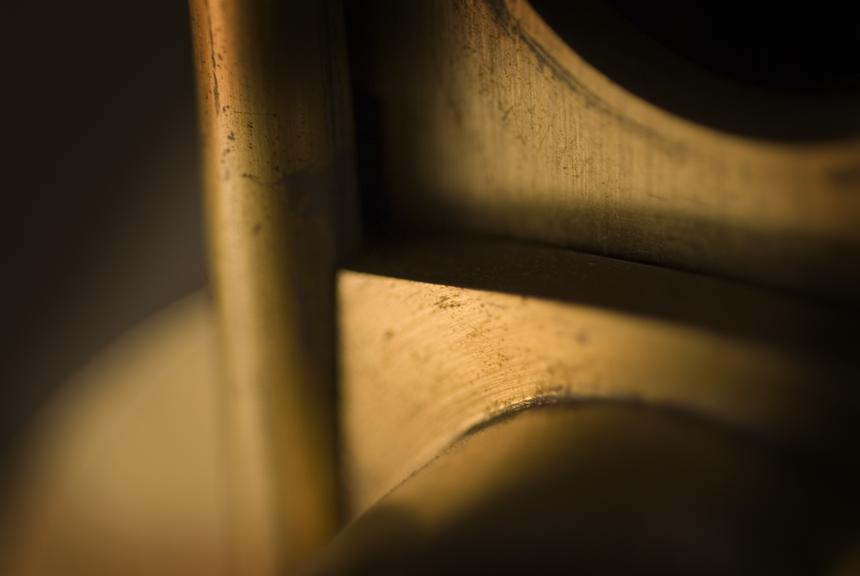The image is a close-up shot capturing a segment of a well-used and aged toilet, characterized by a yellowed and brownish tinge, likely from years of neglect. The focus is on the bottom part of the toilet seat, identifiable by the opening near the top right edge of the frame. Dominating the lower portion of the photograph is the toilet bowl itself. In the center of the image, there is a metal pole, resembling a plunger handle, suggesting an attempt to address a clog. The overall appearance of the toilet evokes the atmosphere of a heavily trafficked, yet poorly maintained public restroom, such as one might find at a truck stop. The photographic clarity is compromised, adding an additional layer of grittiness to the scene.